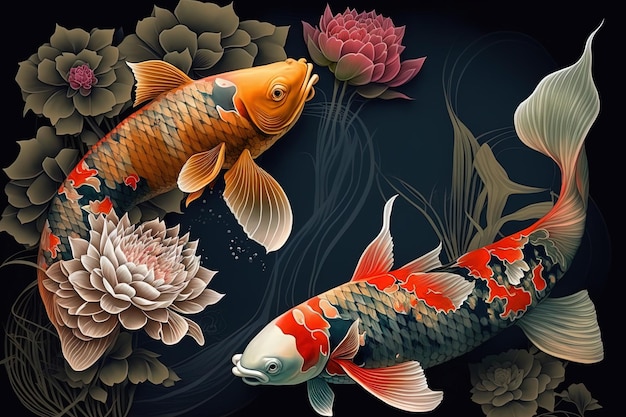In this detailed image, we see two koi fish swimming in a harmonious circular pattern, surrounded by an array of lotuses and aquatic vegetation. The fish in the top left corner displays a striking color gradient, starting with a golden orange head adorned with black eyes and three visible fins. Its body showcases a diamond pattern that transitions from vibrant orange to intense black and red markings towards the tail, which is accented by delicate floral imagery. Surrounding this fish are three pale yellow flowers, one with a pink center, as well as a separate pink flower in the upper section of the image.

The fish in the bottom right is primarily white and grey, with intricate designs of red and grey along its body. This fish has five fins and a long, flowing tail, creating a sense of movement and grace. Bubbles near its lower part enhance the perception of it gliding through water. In addition to the fish, various lotuses in soft hues of white, pink, and magenta surround the scene, with some exhibiting rose and pale yellow tones.

The backdrop is a dark, almost marbled black, creating a dramatic contrast against the vivid colors of the fish and lotuses. Intricate light grey and whiter grey patterns, possibly representing underwater flora, fill the corners and middle section of the image, adding depth and texture to the serene aquatic tableau.